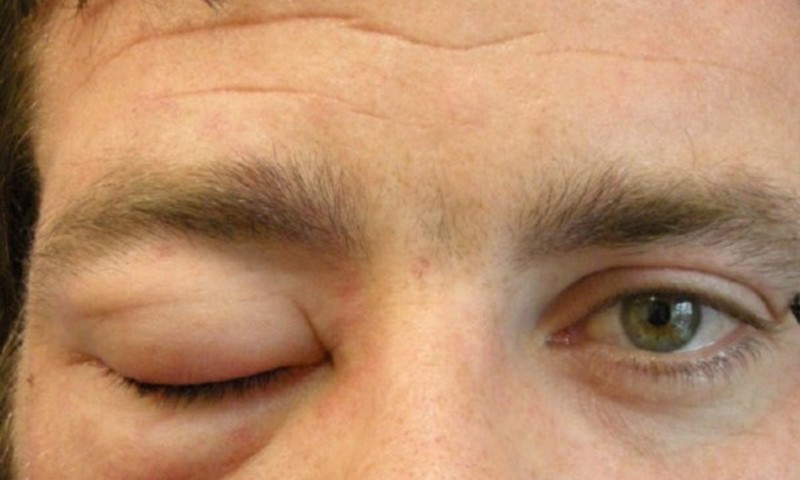This highly detailed close-up image portrays the face of a Caucasian man, primarily focusing on his eyes and a portion of his forehead. His features suggest he is likely in his 30s or 40s, with discernible wrinkles above his eyebrows and noticeable brown hair and eyebrows. The man’s most striking feature is his eye condition: his right eye is open, revealing a greenish-hazel color, while his left eye is closed and evidently swollen, although there is no discoloration or signs of bruising yet. The swelling extends to both the upper and lower eyelids, indicating a recent injury or possibly an infection. The rest of his face is not visible, further focusing the attention on his swollen eyelid and his light eyelashes. Despite his clean complexion, there is a subtle hint of a unibrow, giving a glimpse into his grooming habits. The overall image evokes a sense of mild discomfort or recovery from a recent incident affecting his eye.